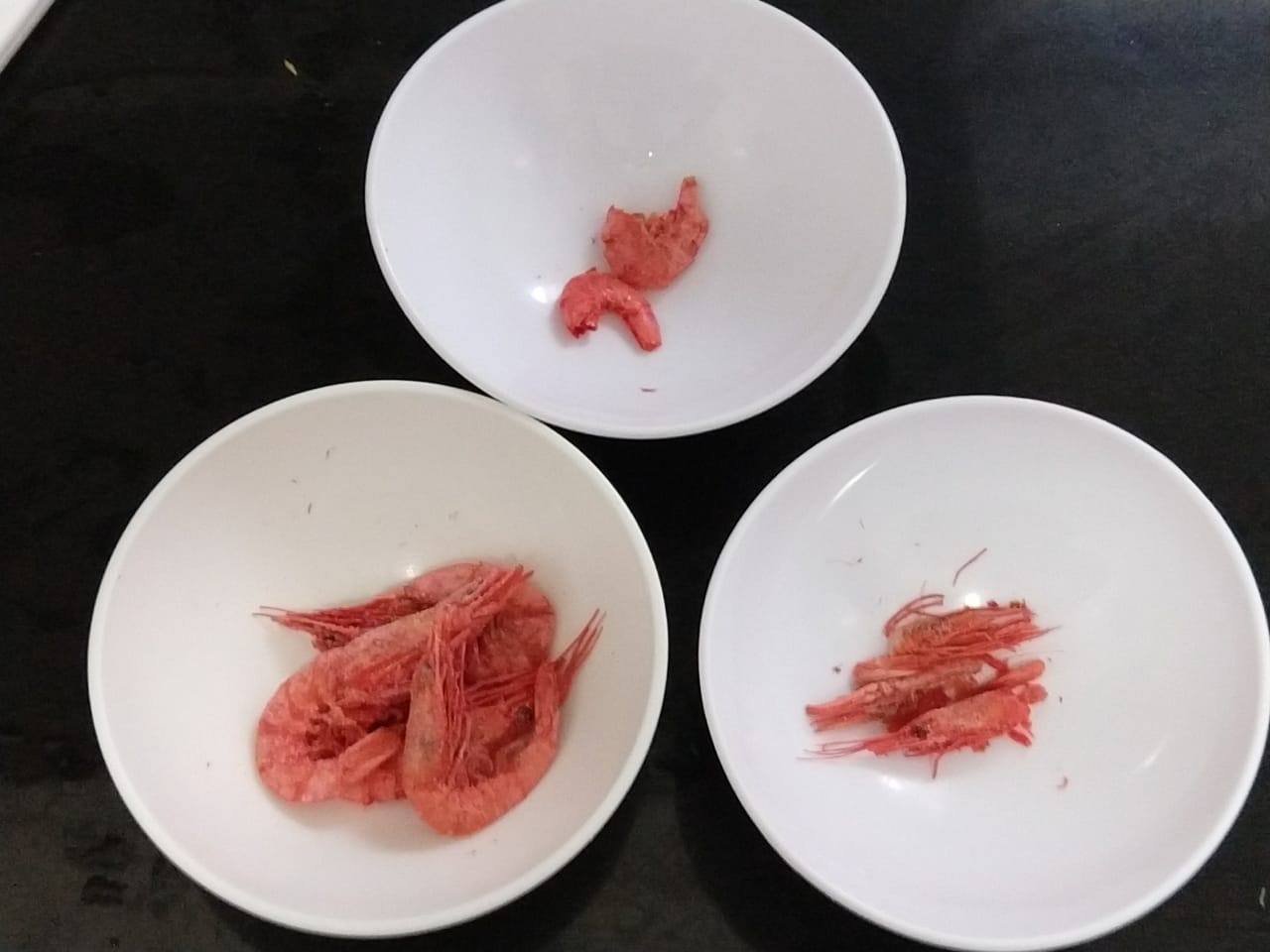In this photograph, we see three white ceramic bowls arranged in a triangular formation on a black table or countertop. The bowls each contain different types of arthropods or invertebrates, primarily shrimp and possibly crawfish, all of which are a light pink color, giving the impression that they are raw. The top bowl, positioned centrally above the other two, contains two small pieces of peeled shrimp, revealing the inner meat. The bottom left bowl appears to hold three to five larger crustacean bodies. Similarly, the bottom right bowl contains about three or four smaller crustaceans, potentially crawfish. The bowls are illuminated by an overhead light, creating a shine on their surfaces. The background behind the bowls is a deep black gradient, adding contrast to the white bowls and their contents. This detailed arrangement captures a careful display of seafood, highlighting the variety and preparation of each crustacean type.